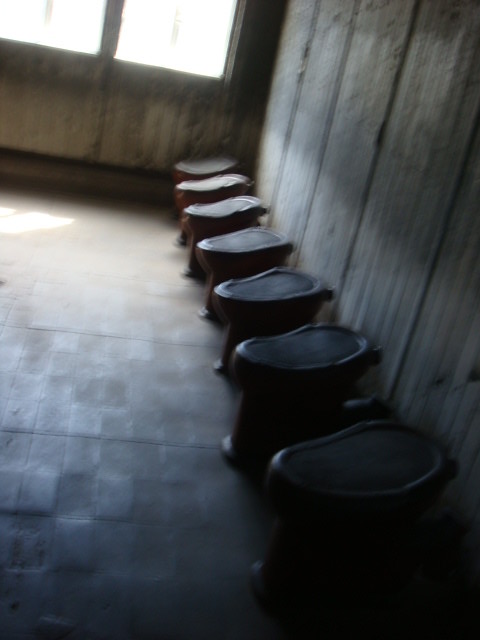This is a slightly blurry, realistic vertical photograph taken in a poorly lit room. The gray floor seems to be ceramic tile or linoleum. Along the right side of the image, there's a brown wooden wall with vertical panels, which continues along the back left of the room, framed by two windows that let in daylight. Against the wooden wall on the right, eight black items are lined up. These items resemble low stools or stylized toilets, characterized by an unusual indented, oval-shaped top without backs or tanks. The room is devoid of people, animals, or mechanical objects.